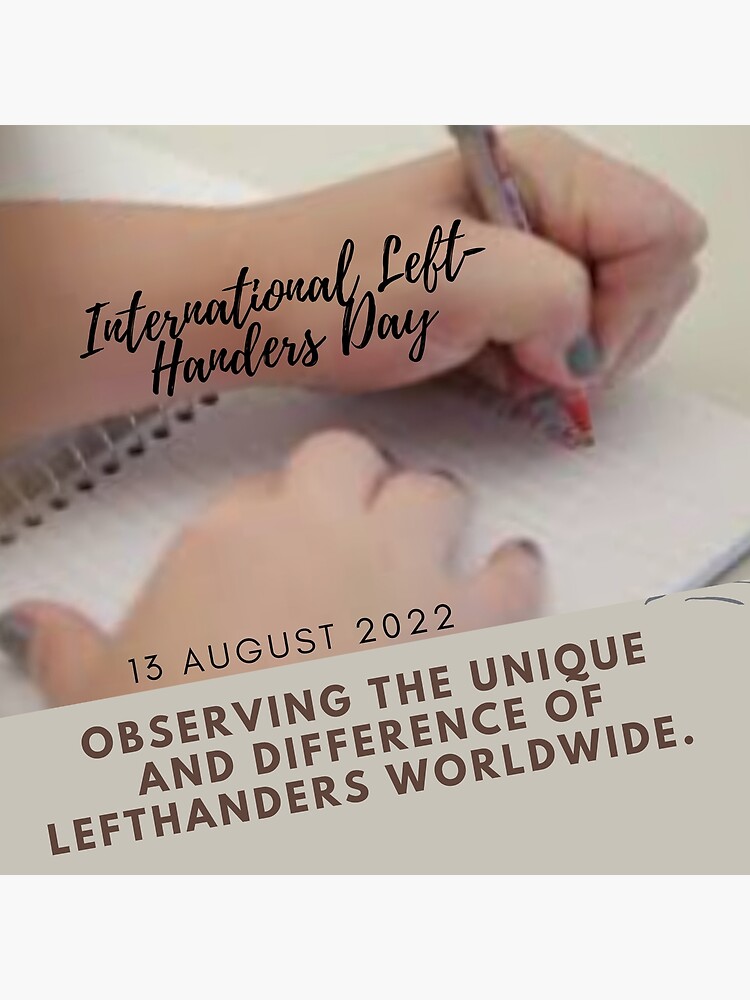This is a close-up photograph of a person writing in a spiral notebook with their left hand, using a red pen. The person's right hand rests on top of the notebook. The writing hand has dark green nail polish. Printed in a cursive font on the arm of the writing hand are the words "International Left-Handers Day," followed by the date "13 August 2022." The words "Observing the unique and difference of left-handers worldwide" are also visible. The image has a beige and brown color scheme and appears somewhat fuzzy, making some details blurry. This image likely serves as a promotional piece celebrating the unique challenges and talents of left-handed individuals.